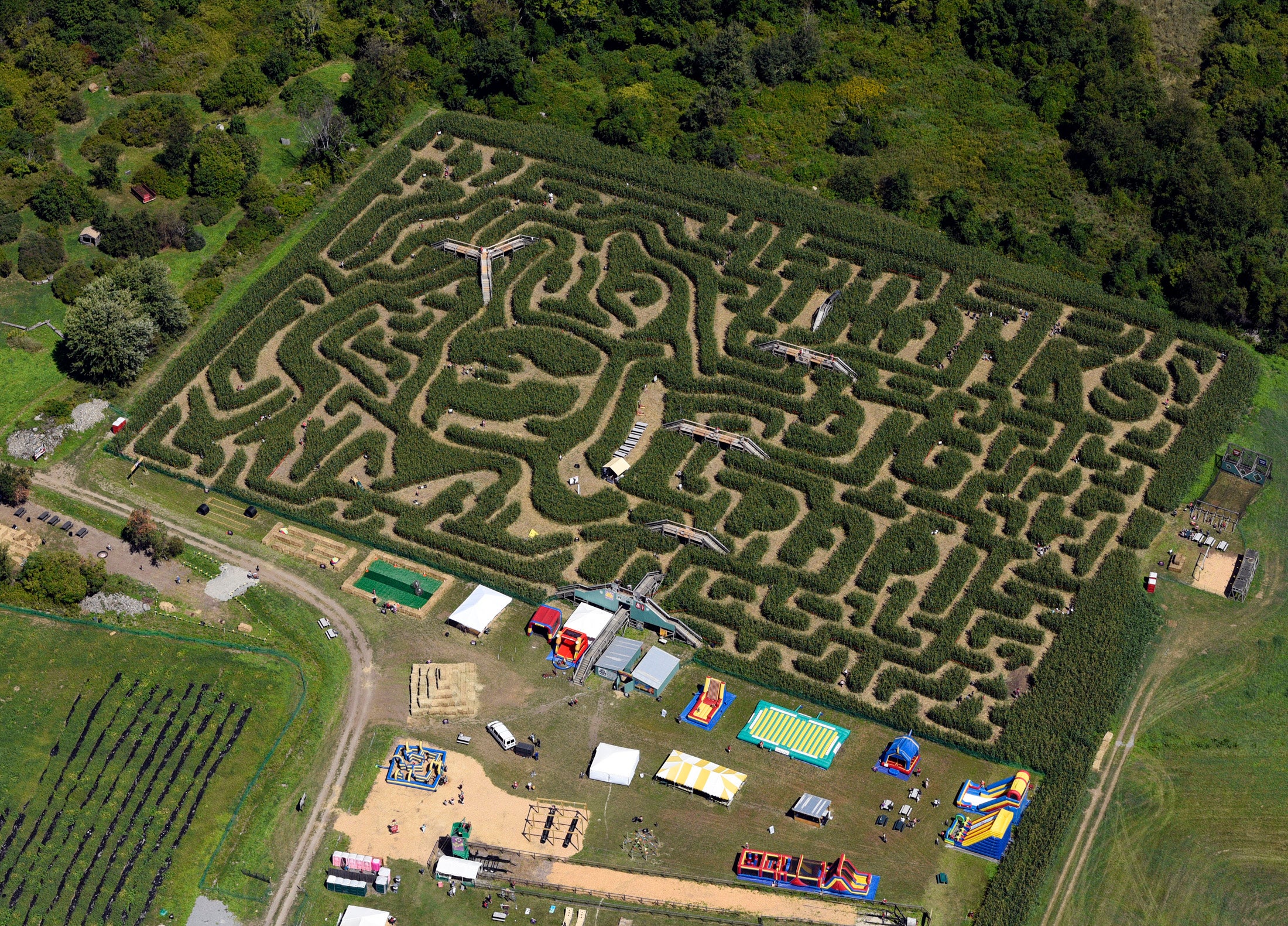This aerial view captures an intricately designed shrubbery maze reminiscent of the one in "The Shining." The centerpiece maze, elaborate and ornate, slants sideways with the words "Thanks Big Poppy" creatively written using the bushes. Surrounding the maze are diverse vibrant colors — shades of green, yellow, brown, black, white, red, blue, orange, and pink. The landscape beyond features hills abundant with verdant trees accented in yellow.

Adjacent to the maze, there are various plots that appear to be designated for farming, evidenced by patches of crops and yellow fields that suggest agricultural activity. There are also visible dirt roads that crisscross through the area, connecting different sections. Scattered throughout, there are several white bridges within the maze and cars parked nearby, although they appear quite small from this distance.

Additionally, the image includes areas dense with green trees, particularly towards the top corners. These tree clusters extend to the middle, providing a green frame around the scene. Below these, there are grassy regions with some containing green crops, interspersed by housing areas and recreational setups like bouncy houses and slides in vibrant colors such as yellow, white, blue, and red. One notable feature is a large blue and white mat and another bouncy structure with a blue bottom along with red and yellow highlights. The houses are mainly white with some having yellowish rooftops. This comprehensive view, likely shot professionally, illustrates a multifaceted landscape blending natural and man-made elements harmoniously. The absence of text within the image enhances its visual storytelling.